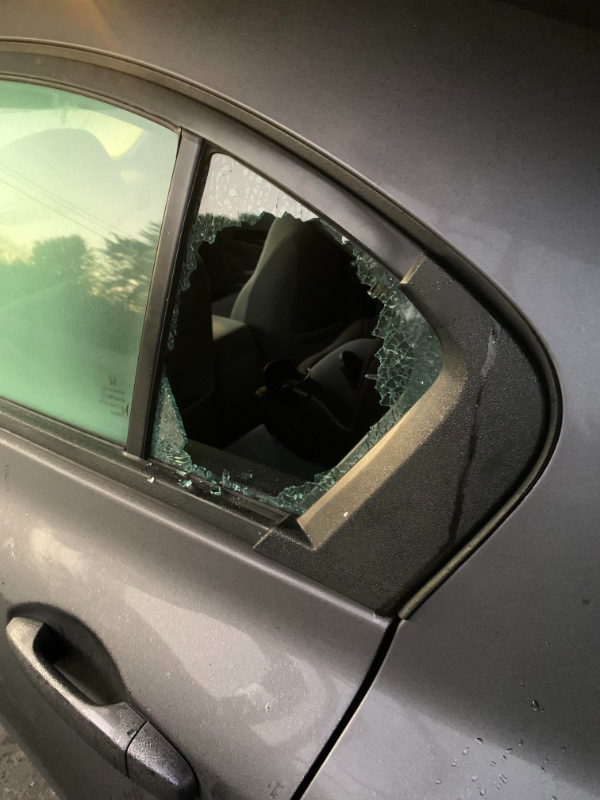In the image, we see a gray car with a broken window. The car's exterior, including the door and the hood, is a shimmery gray color, and the door handle matches this hue. The smaller section of the shattered window reveals that it has a greenish tint, while the larger, green-hued part of the window, enclosed in a gray frame, remains intact. There are small, illegible letters printed on the window. Below, on the bottom edge where the window meets the rubber strip, broken pieces of glass can be seen. The central portion of the window is extensively damaged. The car door appears to have wet spots, possibly from dew or rain, adding to the glossy appearance of the car's body.